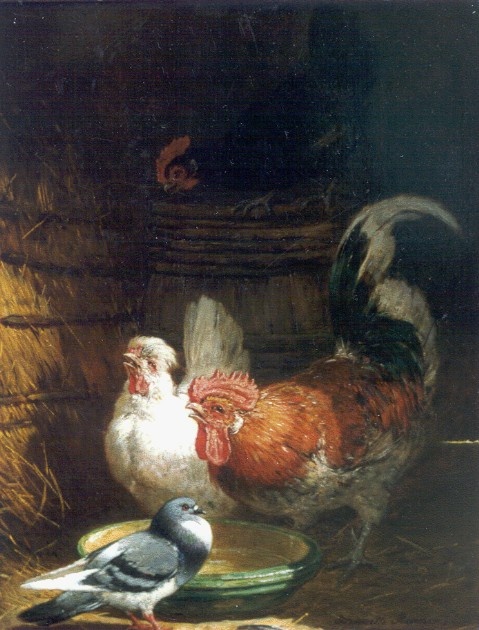This painting, set in a dark barn, vividly captures a rustic scene involving several farm animals. Dominating the left side is a large straw bale, secured with four rope twines, accompanied by an old whiskey barrel beside it. Perched atop the barrel is a black chicken with a striking red crown and its tail feathers raised high. On the ground, near a large, shallow green bowl possibly containing water or chicken feed, stands a gray pigeon with distinctive black stripes on its wings and orange feet. This pigeon seems out of place amongst the farm animals, which include a large rooster with a red body, a black and white tail, and prominent red wattles under its beak. Beside this rooster is a white chicken with a puffy head. The overall depiction brings to life the textured details of the hay-strewn floor and the contrasting colors and characteristics of the barnyard birds.